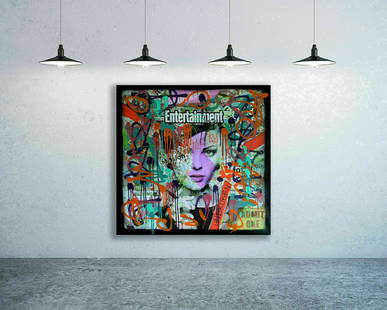The image showcases a large, square painting hanging indoors on a white wall, with a sturdy black frame encasing it. The focal point is a partly visible woman's face gazing forward, centered beneath the word "ENTERTAINMENT" inscribed across the top, giving it the appearance of a stylized magazine cover. Surrounding the central figure are vibrant, abstract splashes of color in orange, purple, and blue, contributing to the dynamic composition. In the lower right corner, a small yellow "admit one" token can be discerned, adding an intriguing detail. The painting appears to have areas where the paint looks freshly applied, giving a fluid impression. Four overhead black lamps, suspended by thin cords from the ceiling, cast focused light onto the painting, enhancing its prominence against the backdrop of the grayish-beige floor below. The entire area is devoid of people, imparting a quiet, contemplative atmosphere to the scene.